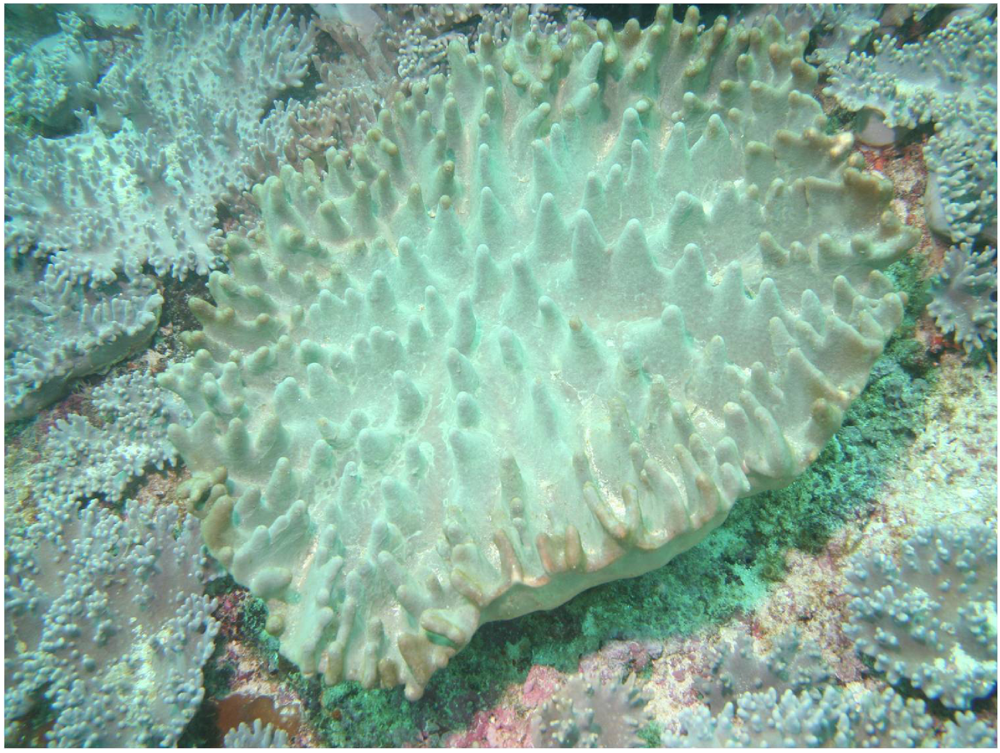This rectangular image, wider than it is tall, vividly captures an underwater scene featuring what appears to be an array of sea creatures or sea plants, blending seamlessly with their coral surroundings. The centerpiece of the image is a striking sea entity, predominantly whitish-green, accented with light brown tips around its edges. Its surface exhibits a textured pattern reminiscent of tall mountain ranges or simple pine tree drawings, composed of rounded spikes that, while not sharp, suggest a potential deterrent to predators. This central figure is irregularly shaped, skewing towards an oval but tapering into slight points at the bottom, creating a unique silhouette.

Surrounding this central feature are numerous smaller, textured fragments in hues of whitish blue and gray, contributing to the complex and varied landscape. A greenish silhouette enhances the lower contours of the central organism, adding to the vibrant, multi-colored palette that includes splashes of pinks and yellows. The brightness of the image suggests it was taken in a well-lit underwater environment, allowing the rich colors and details of this undersea tableau to be clearly visible.